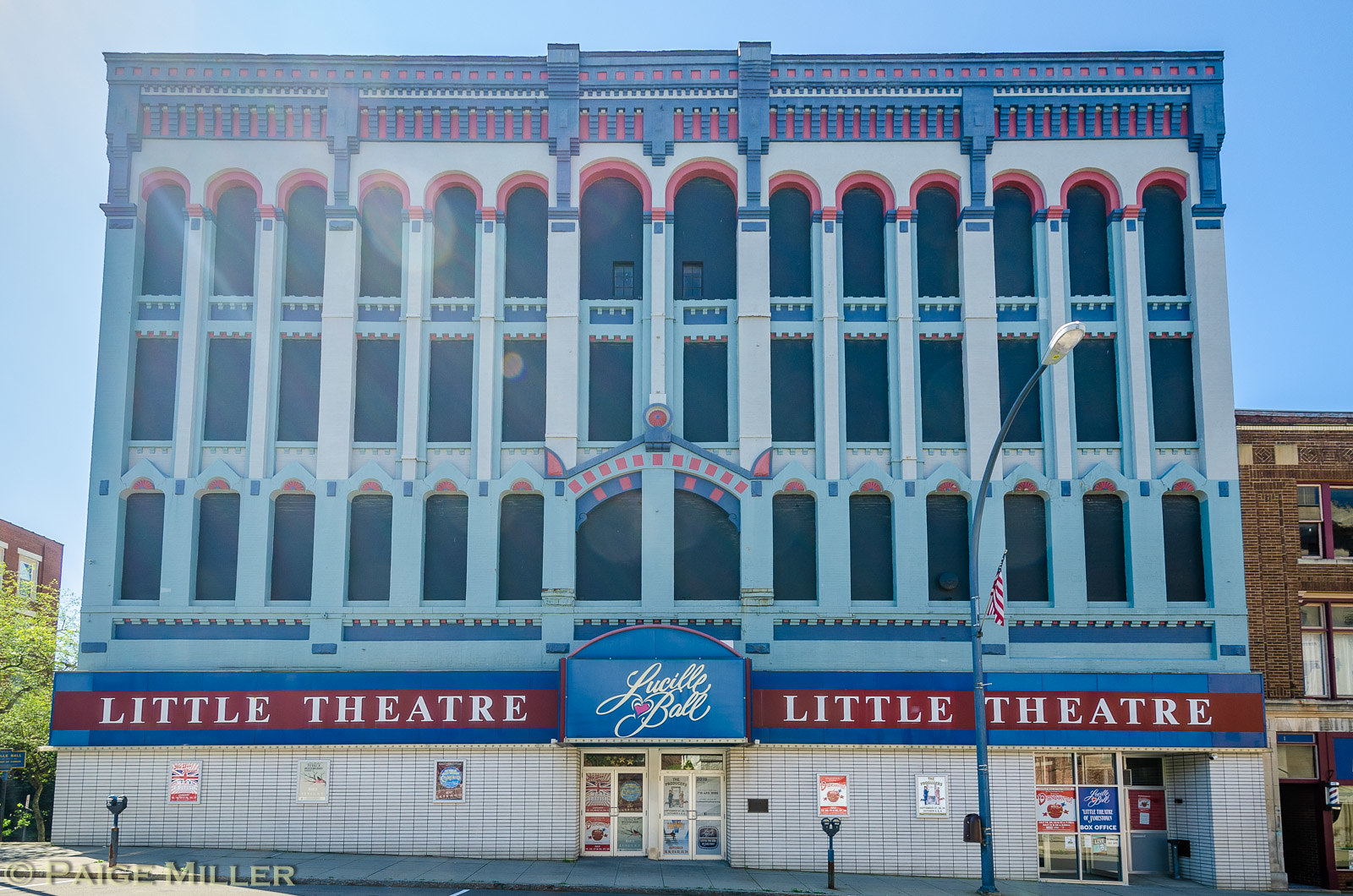This photo captures a prominent four-story theater building, predominantly white with striking red and blue decorations. The vibrant blue roof contrasts with red inlays in the flat crown molding at the top. The façade features tall, black arched windows with red accents on the upper floors and white pillars with blue in-between.

The bottom story is characterized by a strip of white tiling and glass doors framed in silver, positioned centrally and to the far right. Above, a large blue awning bearing the name "Lucille Ball" shelters the main entrance. Beneath it is a red banner, stretching across the front, emblazoned with "Little Theatre" in white text. This banner is repeated near each side of the entrance.

The building is flanked by light posts and parking meters, grounding its presence as the centerpiece among smaller buildings to the left and right. The iconic design and notable references make it unmistakable as the Lucille Ball Theatre, a memorable landmark.